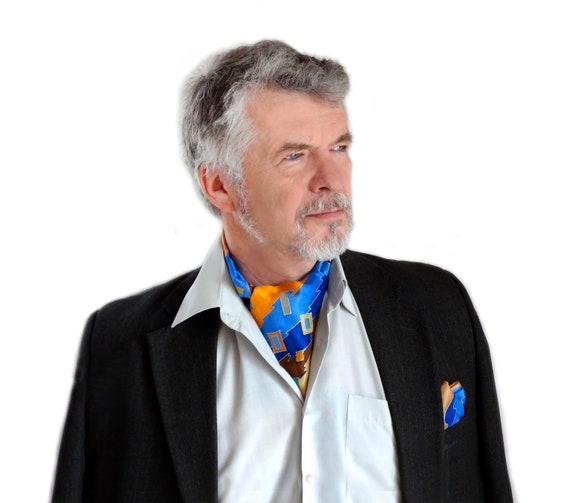This is a detailed portrait of a distinguished, elderly gentleman, whose appearance exudes a sense of familiarity. His body faces directly towards the camera, while his head is turned slightly to his left, giving the composition a subtle dynamism. He sports a full mane of gray hair and a matching beard that's neatly kept, complemented by long, distinguished sideburns. His attire is impeccable: he is clothed in a black suit coat with a crisply pressed white shirt beneath. Notably, he dons a cravat adorned in a rich tapestry of blues, orange, dark blue, and brown hues, a color scheme that's thoughtfully echoed in the handkerchief peeking out of his coat pocket. His piercing blue eyes convey a sense of earnestness and depth, adding further to the portrait's sense of gravitas and character.